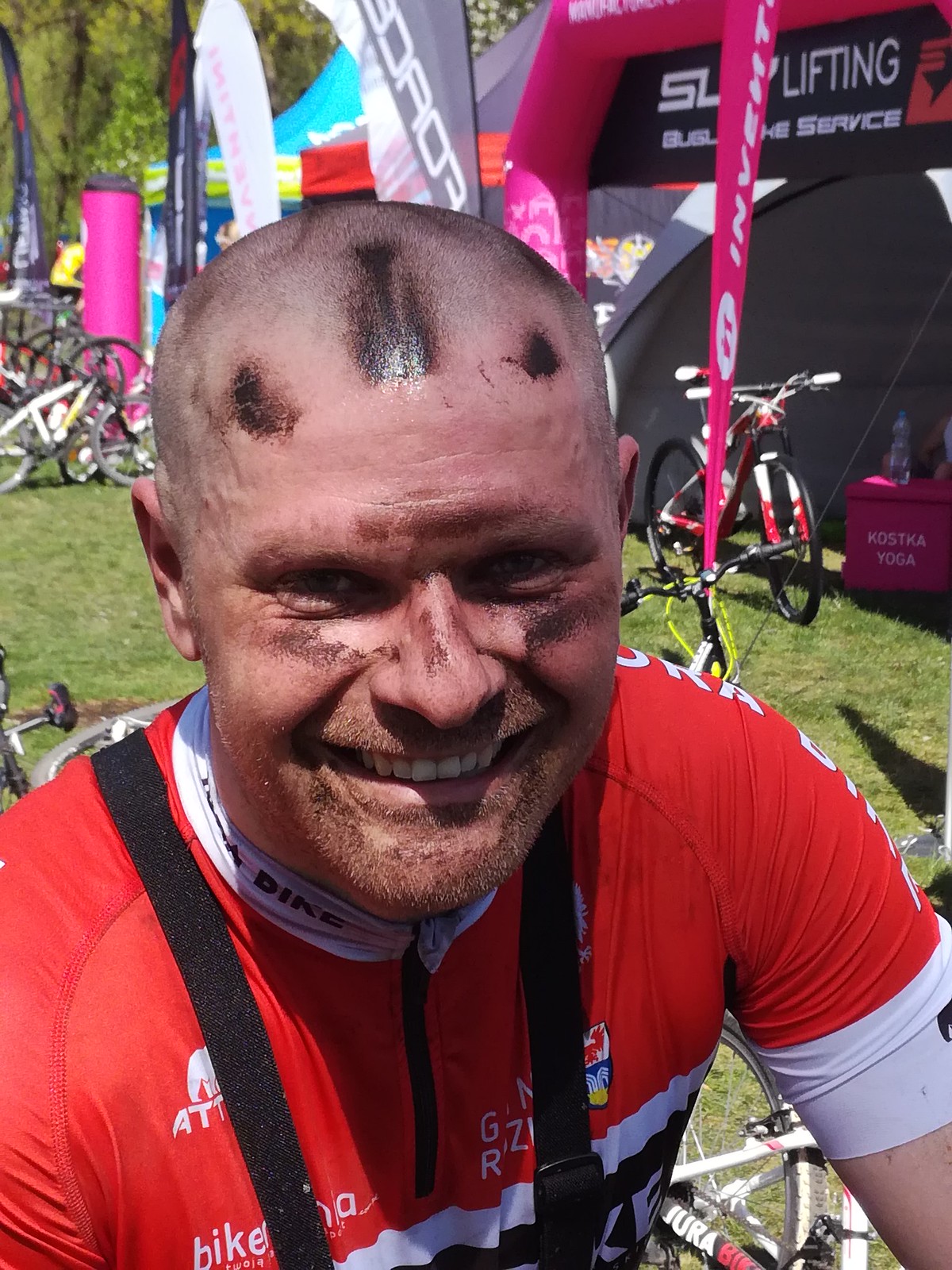The image depicts a middle-aged, Caucasian man with a closely shaved head, presumably just after completing a bicycle race. He is smiling warmly despite having grease and dirt smeared across his head and face, most prominently in the middle and top of his head. His face is covered with stubble on his top lip and chin. He wears a red and white cycling jersey featuring black shoulder straps and white letters. Only his upper chest and head are visible. The background is a vibrant scene, filled with numerous bicycles, booths with brightly colored banners and signs, and some trees. The man seems to be straddling a bicycle, although only a part of a bike is visible just behind him. The entire setting rests upon a grassy field.